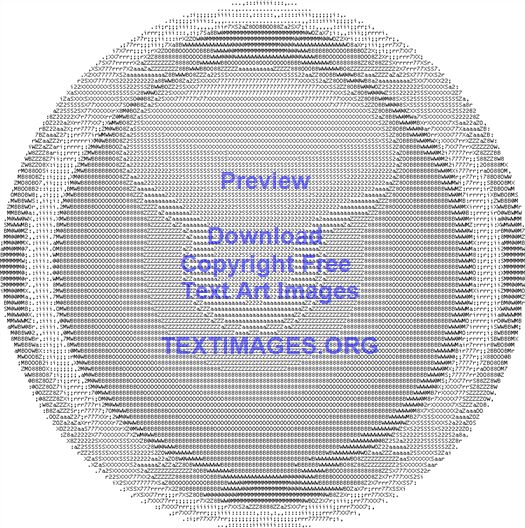The image is a highly detailed graphic design of a circular button against a plain white background. The circle itself is predominantly black and white, composed of numerous small letters and numbers, creating a textured and pixelated effect. From a distance, the circle appears whitish silver or gray with white highlights around the edge, resembling a plate. The very center of the circle features a darker hue with a slightly indented look, enhancing the button-like appearance. Prominently displayed in a royal blue or bluish-purple Arial font, the text reads: "Preview, Download, Copyright Free Text Art Images," followed by "textimages.org" in bold at the bottom of the circle.